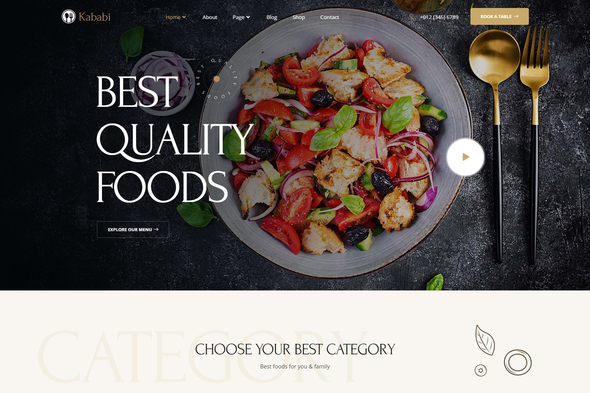Online Platform for Vegetarian Cuisine: An inviting web page of "Kebabi" showcasing their commitment to the "Best Quality Foods" in bold, white uppercase letters against a sophisticated dark background. At the center, a meticulously arranged salad graces a dinner plate, featuring vibrant red peppers, crisp onions, juicy tomatoes, and fresh lettuce, enhanced with what appears to be some breaded components. 
To the right of the plate, an antique silver fork and spoon with sleek black handles add a touch of elegance. 
The top navigation menu of the website includes tabs: 'Home,' 'About,' 'Blog,' 'Shop,' and 'Contact,' providing easy access to explore various sections. Beneath the prominent slogan, a small black box with white uppercase letters invites visitors to "Explore Our Menu," promising a delightful culinary journey through vegetarian fare.